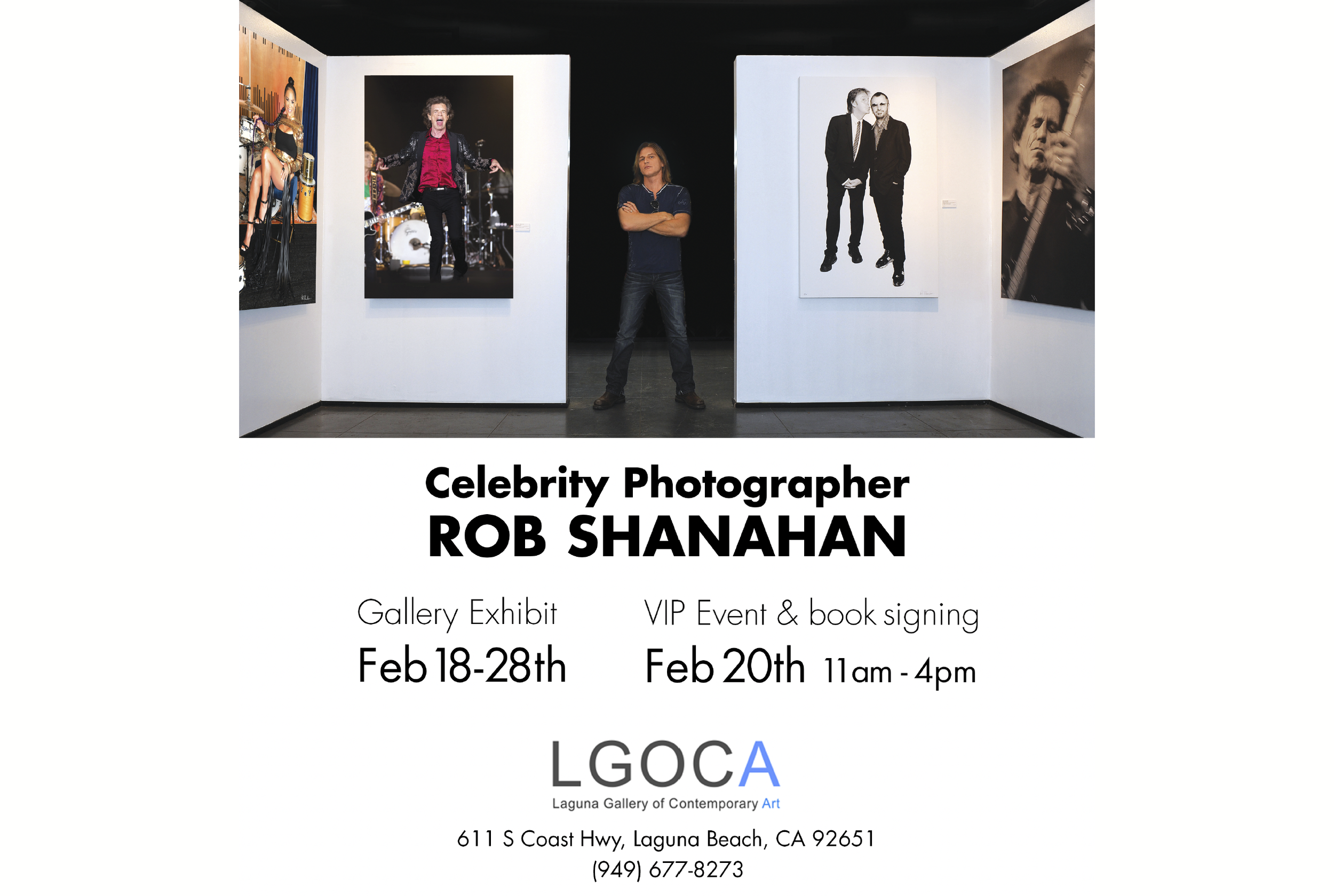The advertisement for a photography exhibit, prominently set against a white background, features a compelling photograph at the top of the page. The photograph showcases celebrity photographer Rob Shanahan, a light-complected man with shoulder-length brown hair, standing confidently with his arms crossed between two white wall partitions that display his works. He is attired in a blue short-sleeve t-shirt, dark blue jeans, and brown shoes, emphasizing his casual, approachable demeanor.

Flanking him on both sides are pairs of his poster-sized photographs. On the left partition, the top image portrays a woman with short black hair in a bun, seated against an orange-red background. She is dressed in a black tank top with a beige over-shirt, complementing her long legs. The bottom image features a man in a black jacket, red undershirt, black pants, and black shoes, standing in front of a substantial drum set. The right partition includes an image of two men whispering, one in a black suit with a white shirt and tie, the other in a black tuxedo with glasses. The bottom photograph is a close-up of a bassist, fingers poised on the instrument, against a predominantly black and gray backdrop.

Below the central photograph, in bold black letters, is the text: "Celebrity Photographer Rob Shanahan." To the left beneath this is the announcement: "Gallery Exhibit, February 18-28." To the right, it reads: "VIP Event and Book Signing, February 20, 11am-4pm." At the very bottom, the advertisement details: "LGOCA - Laguna Gallery of Contemporary Art, 611 South Coast Highway, Laguna Beach, California 92651. Phone: (949) 677-8273." This comprehensive caption encapsulates every essential detail, providing a vivid description of the exhibit's visual and text elements.